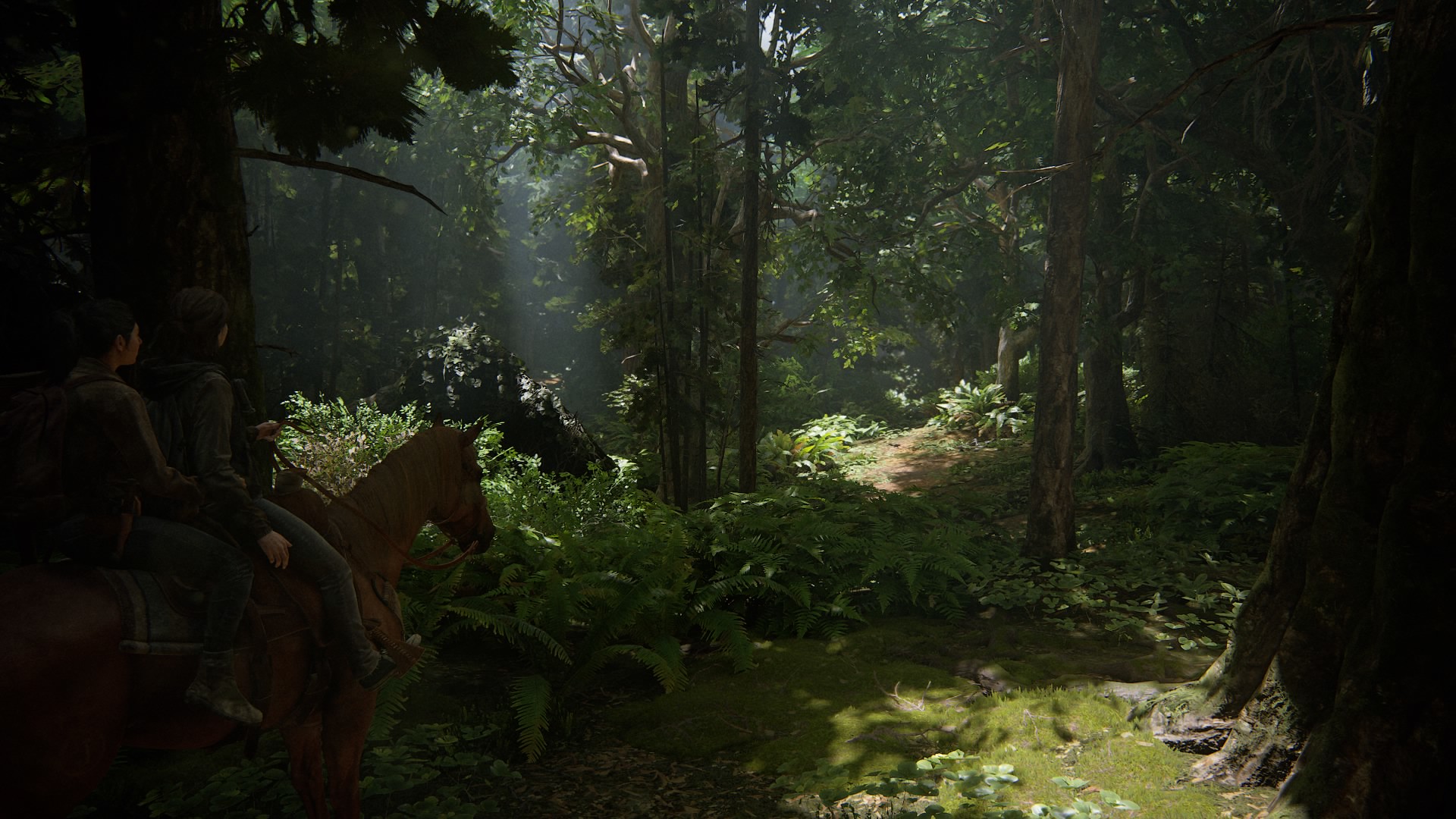In this forest scene painting, the image predominantly features a dense and vibrant woodland area with abundant greenery and towering trees. Sunlight pierces through the canopy, casting illuminated patches onto the forest floor and creating an interplay of light and shadows. In the far bottom-left corner, a brown horse with a saddle stands, carrying two riders—a girl in front and a boy behind. The girl has long black hair flowing past her shoulders, while the boy's hair reaches the length of his neck. Both riders are clad in long pants and long shirts, possibly sweatshirts, hued in shades of gray. The composition suggests they are venturing into the forest, which lacks a discernible path but shows signs of trodden areas dotted with various plants and bushes. Adding to the rich tapestry of nature, there are clusters of white flowers and other colorful vegetation nearby, with roots and tree trunks partially visible amidst the sunlit grass in the center of the scene.